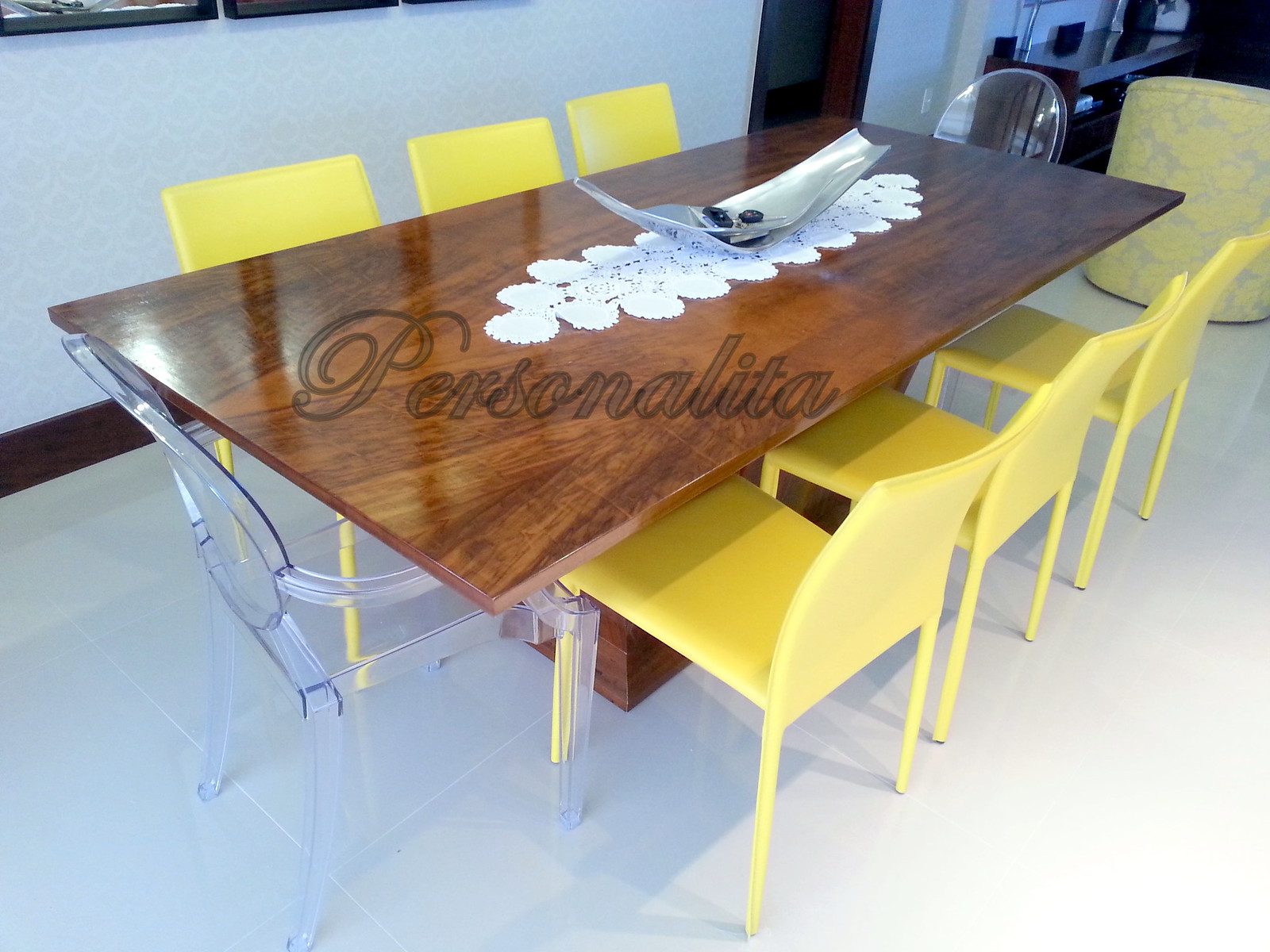This detailed photograph depicts an elegant indoor setting, likely part of either a business space or someone's home dining room. Central to the image is a long, polished wooden table with a smooth, lustrous surface and sturdy legs made from the same dark wood. Adorning the middle of the table is a delicate white lacy doily, atop which rests an abstract, silver metal bowl that might be holding a set of keys. The table is surrounded by a total of eight chairs: three bright yellow armless chairs flanking each of the table's long sides and two transparent, clear plastic chairs positioned at each end. The room's flooring is comprised of shiny white porcelain tiles, so reflective that the chairs and the table are mirrored upon it. The walls match the floor in their clean white color. In the top right corner of the image, there is a light gray chair with a vibrant yellow floral design. Additionally, a black TV stand, potentially holding a speaker, can be seen against the white wall. These details come together to craft a harmonious and stylish atmosphere in the room.